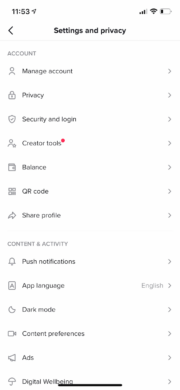Caption: "A detailed view of a tablet displaying a settings and privacy menu screen. The top-left corner shows a timestamp '113053,' while the top-right corner displays cell signal bars, Wi-Fi signal strength, and a low battery icon. Below this, a left-facing arrow is labeled 'Settings and Privacy.' The main content area is a left-justified list of options, each with corresponding right-facing arrows: 'Account,' 'Manage account,' 'Privacy,' 'Security,' 'Creator tools' (with a tiny red dot above the 'S'), 'Balance,' 'QR code,' 'Share profile,' followed by sections 'Content & Activity,' 'Push notifications,' 'App language' (set to English), 'Dark mode,' 'Content preferences,' 'Ads,' and 'Digital well-being.' The list is in a black font that appears gray due to poor resolution, and the background is a mix of gray, black, white, and a single red dot. This menu fills the entire tablet screen, appearing larger than it would on a phone."